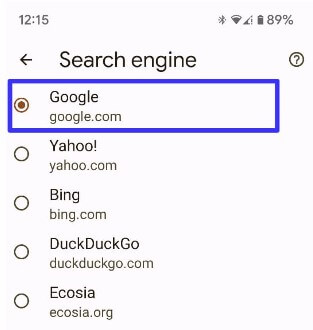This is a screenshot of an admin page displayed on a mobile phone, captured at 12:15 PM. The status bar at the top indicates various icons: a Bluetooth symbol, a Wi-Fi signal at approximately 75% strength, a cellular signal at about 50% strength, and a battery level at 89%.

Below the status bar is a navigation bar featuring a back arrow on the left and a question mark encased in a circle on the right. The main content of the screen allows the user to select a default search engine from a list of five options, each with a corresponding radio button for selection. Only one option can be selected at a time.

The first option, highlighted with a purple border featuring sharp corners, is Google (google.com) and is currently selected. The second option is Yahoo! (yahoo.com), followed by Bing (bing.com). The fourth option is DuckDuckGo (duckduckgo.com), and the final option is Ecosia (ecosia.org).

The rest of the screen remains white, with no further information displayed. The image is cropped just below the search engine options, excluding any potential navigation buttons or additional menus that may reside at the bottom of the page.